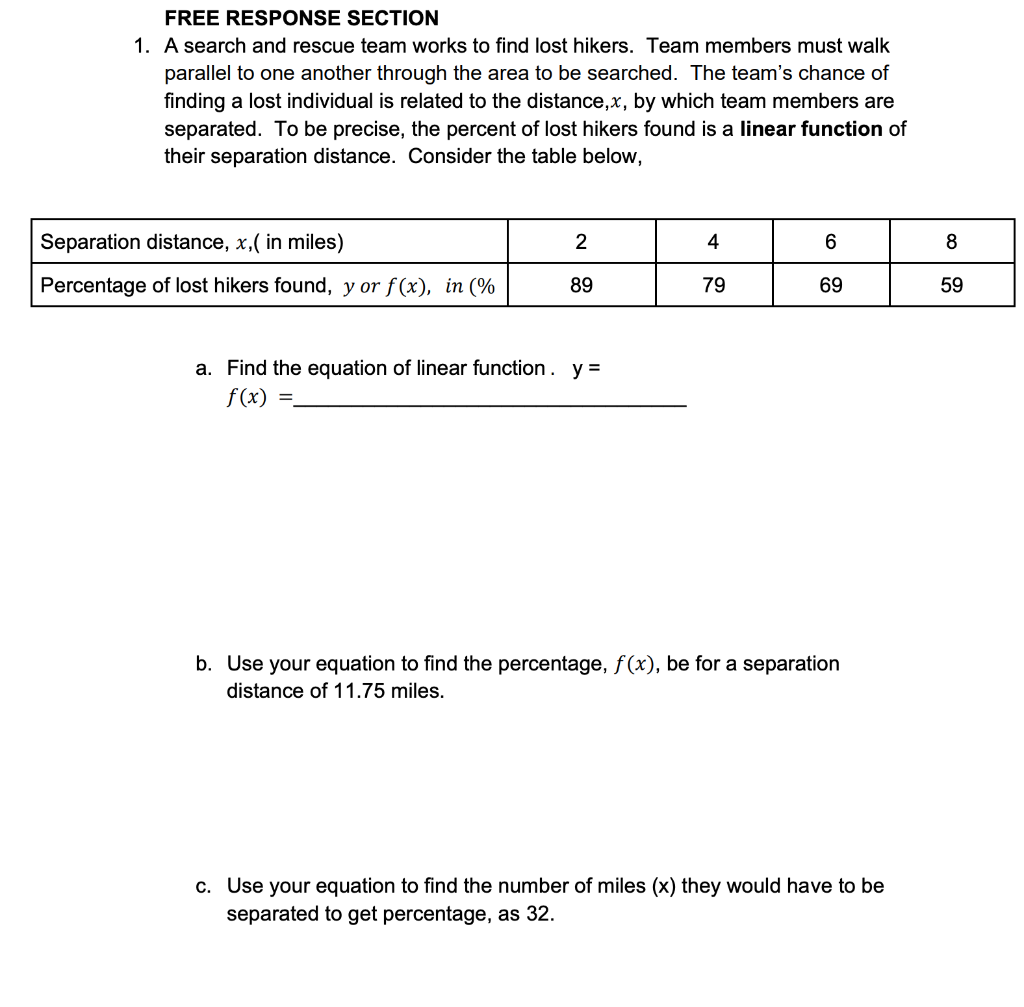The image shows a black-and-white, portrait-oriented math worksheet, specifically the first problem in the free response section. The problem presents a scenario involving a search and rescue team working to find lost hikers. It describes that team members walk parallel to each other and that the chance of finding a lost individual is a linear function of their separation distance, denoted as X. A table below this explanatory text lists separation distances in miles (2, 4, 6, 8) in the first row and the corresponding percentage of lost hikers found (89%, 79%, 69%, 59%) in the second row. The problem is sectioned into three parts labeled A, B, and C, each requiring the student to use the table to solve related equations. There is ample space provided under each part for calculations.